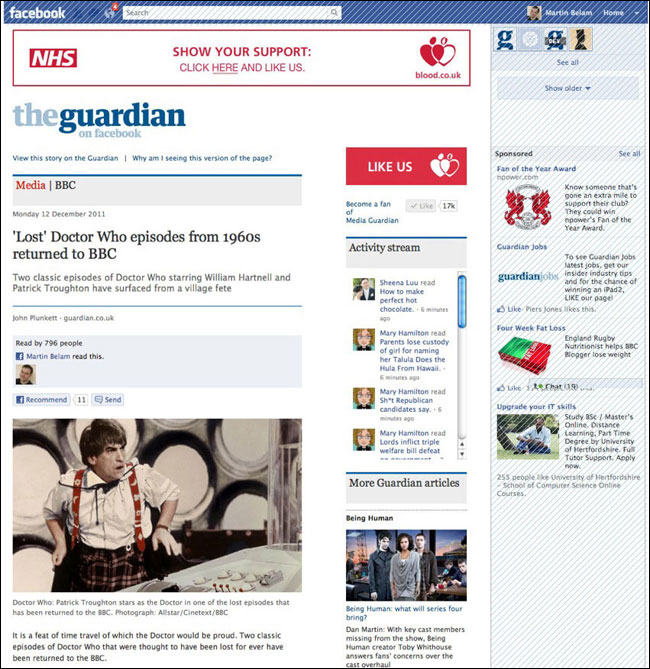A detailed screenshot from a Facebook page displays an article from The Guardian. At the top of the screenshot, there's an advertisement that reads, "NHS, show your support, click here and like us," with a URL pointing to blog.co.uk. Below the ad, the Facebook interface indicates that the article is hosted on The Guardian's Facebook page, featuring an option to view the story directly on The Guardian's official site. Users are also provided with a link indicating why this version of the page is being shown.

Dated Monday, December 12th, 2011, the post highlights a significant media discovery: two lost episodes of the classic 'Doctor Who' series from the 1960s have been returned to the BBC. The episodes feature the iconic Doctors played by William Hartnell and Patrick Troughton and were reportedly found at a Village Fete by Josh Plunkett. The article, read by 726 people, is authored by Martin Bellum. It also includes a photograph credit to Alastair/Clientech/BBC, displaying a scene with Patrick Troughton as Doctor Who from one of the recovered episodes.